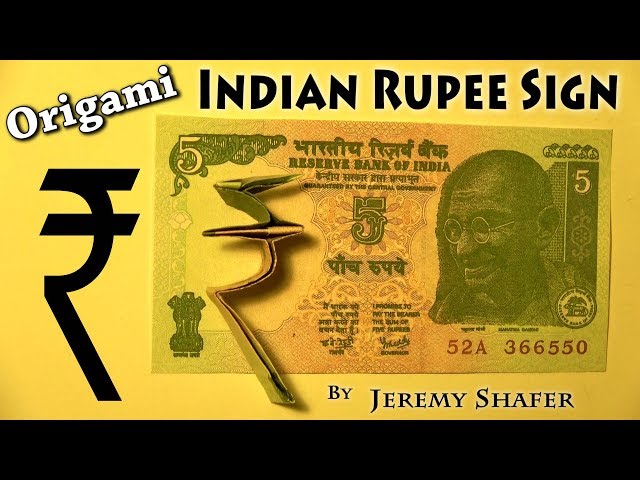The image features a detailed composition set against a black background. Central to the image is a prominent yellow panel. At the top of this panel, "Indian Rupee Sign" is inscribed in bold black letters. Diagonally across the yellow panel, the word "Origami" appears in white letters on the left side. 

Below this, a black rupee sign is visible on the left side of the panel. Positioned in the center of the image is a real 5 Indian Rupee banknote, seemingly adhered to the yellow surface. This banknote displays the face of Mahatma Gandhi prominently on the right, alongside the text "Reserve Bank of India." The note's coloration is predominantly green with a pinkish-red center and includes various inscriptions in Hindi.

At the bottom of the yellow panel, the caption "By Jeremy Schaefer" is noted, marking the creator of this artwork. The overall arrangement juxtaposes the bright yellow panel and the detailed banknote against the stark black background, adding a striking visual contrast to the composition.